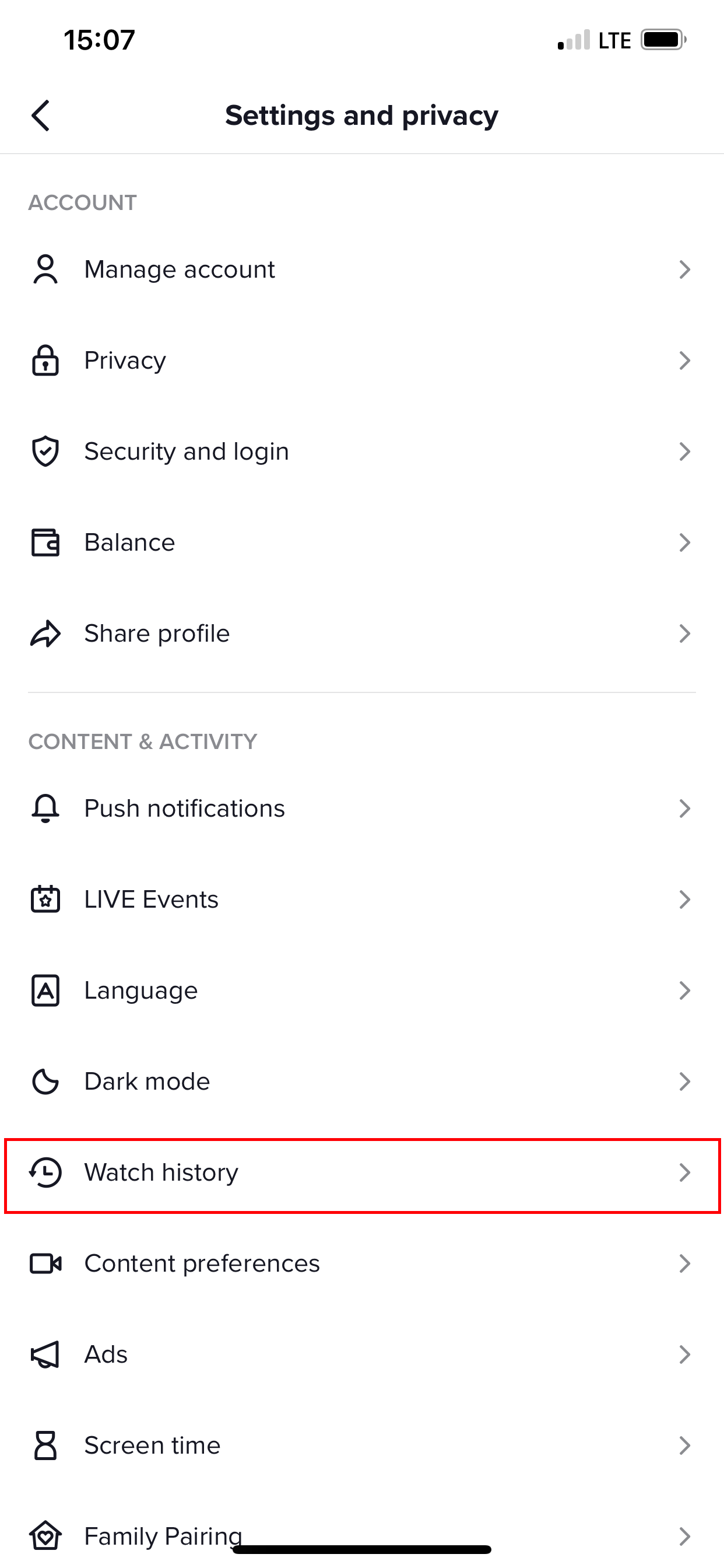### Detailed Caption for App Settings and Privacy Screenshot

The image displays a screenshot of the "Settings and Privacy" section of an app, captured at 15:07. In the top-left corner, the time "1507" is clearly shown. Moving to the top-right, the status bar shows a single filled bar indicating low signal strength, followed by "LTE" beside it. Adjacent to these, the battery icon appears.

The "Settings and Privacy" screen is divided into two main sections. The first section is labeled "Account" and includes several options: "Manage Account", "Privacy", "Security and Login", "Balance", and "Share Profile". 

Below this, there is a section titled "Content and Activity". Here, various options are listed: "Push Notifications", "Live Events", "Language", "Dark Mode", "Watch History", "Content Preferences", "Ads", "Screen Time", and "Family Pairing". Notably, the "Watch History" option is highlighted with an outline in a reddish-orange color reminiscent of a car's paint.